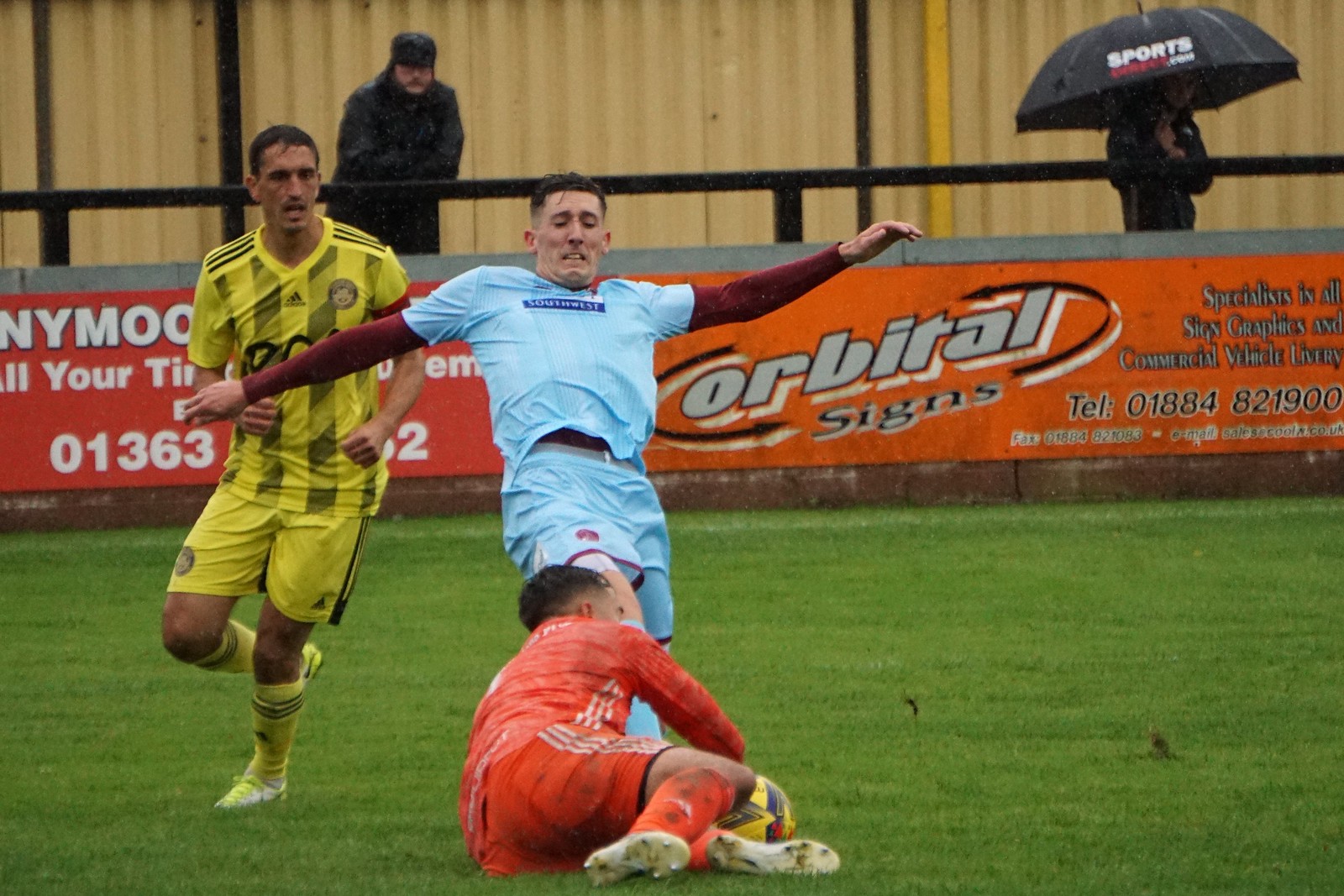In this detailed scene of a soccer game on a rain-soaked, green field, three players are intensely engaged in the action. The player in the orange uniform lies on the ground on his left side, covered in mud, with his orange socks pulled up to his knees. Nearby, a soccer ball sits prominently on the grass. A player in a blue uniform with a red long-sleeve undershirt is poised to kick the ball, though the angle makes it seem he might accidentally kick the fallen player. In mid-stride, a player in a yellow uniform runs towards the scene, his right leg and foot suspended in the air. The game appears to be set in rainy conditions, as evidenced by a black umbrella held by a spectator in the upper right area and a barrier with advertisements behind the players. Another spectator stands behind the barrier, adding to the atmosphere of a closely watched game.